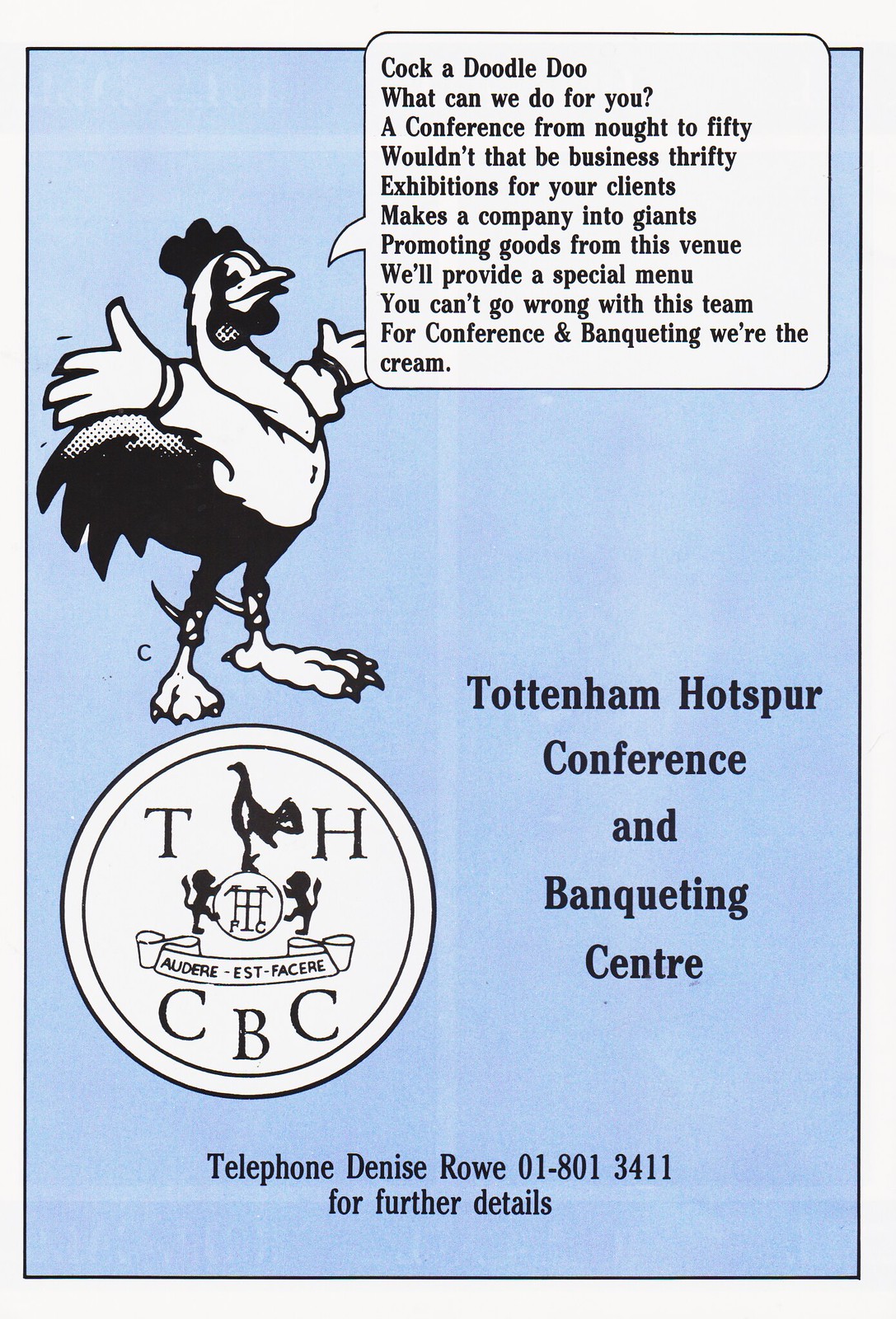This detailed advertisement, likely from an older magazine or a soccer program, promotes the Tottenham Hotspur Conference and Banqueting Center. It features a light blue background with a black and white circular logo that includes the initials THCBC, a rooster, and two small lion silhouettes. Central to the design is an illustrated anthropomorphic rooster holding out its hands and exclaiming in a speech bubble: "Cock-a-doodle-doo, what can we do for you? A conference from naught to 50, wouldn't that be business thrifty?" The advertisement also highlights the center's services, boasting, "Exhibitions for your clients makes a company into giants promoting goods from this venue. We'll provide a special menu; you can't go wrong with this team. For conference and banqueting, we're the cream." The contact details at the bottom encourage potential clients to call Denise Rowe at 01-801-3411 for further information.